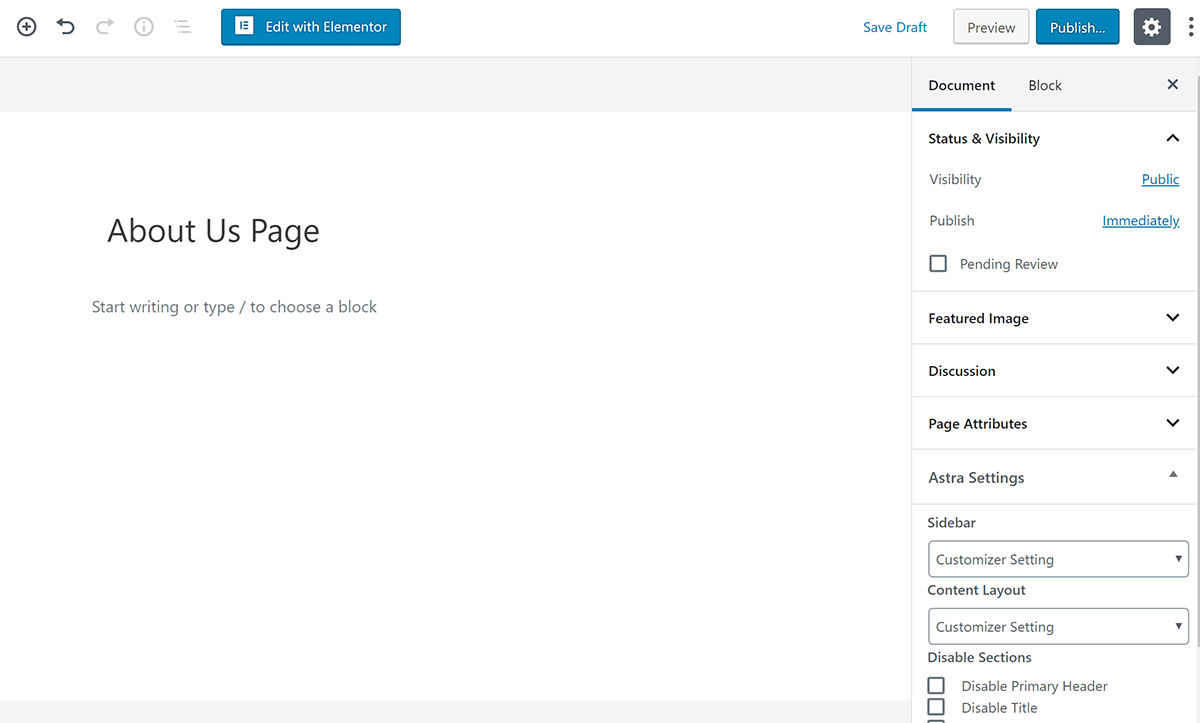The image depicts the user interface of a web page builder, possibly Elementor. In the top left corner, there is a circular button with a plus sign inside it, followed by a highlighted redo arrow. Adjacent to it, there is a grayed-out redo arrow pointing to the right. Additionally, there is a grayed-out circular icon featuring an exclamation mark, alongside a three-line menu icon. There is a prominent green button labeled "Edit with Elementor."

On the right-hand side of the interface, there is a "Save Draft" button, followed by a gray "Preview" button, and a blue "Publish" button. Next to these, there is a settings cog icon in dark gray and a button comprising three vertical dots.

Below these controls, the interface displays two tabs: "Document," which is underlined in blue, and "Block," which can be closed using an adjacent 'X'. The "Status and Visibility" section features a drop-down arrow, indicating further options. Within this section, "Visibility" is highlighted in blue as "Public," and "Publish" is also highlighted to denote immediacy. Additional options such as "Featured Image," "Discussions," "Page Attributes," "Asterisk Settings," "Sidebar," "Content Layout," and "Disabled Sections" are also present on the right-hand side.

Central to the interface is an "About Us" page, prompting the user to begin writing or to type a forward slash to choose a block for content creation.